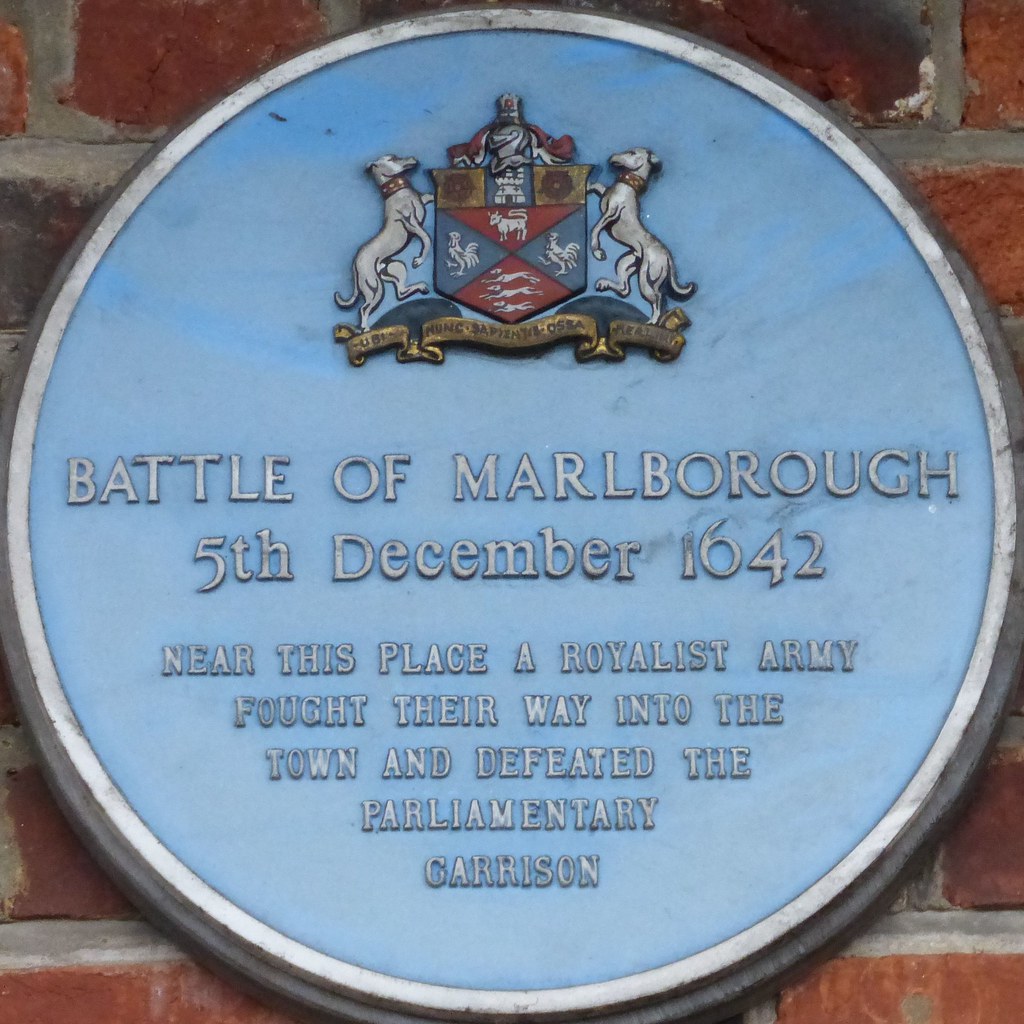The image showcases a slightly weathered circular seal mounted on a red brick wall, with gray mortar between the bricks. The seal itself is primarily light blue with a silvery-gray border, which appears somewhat tarnished and dirty. At the top of the seal is an ornate shield flanked by two identical greyhounds, each dog standing with one paw on the shield. These dogs wear red collars, and the shield displays various sections in red, yellow, and blue, including depictions of racing dogs, an ox, a chicken, and possibly another rooster. Above the shield is a crown, while a gold banner with indistinct writing waves at the bottom. The central text on the seal reads: "Battle of Marlborough, 5th December 1642." Below this, in smaller, capitalized, silvery-gray letters, it states: "NEAR THIS PLACE A ROYALIST ARMY FOUGHT THEIR WAY INTO THE TOWN AND DEFEATED THE PARLIAMENTARY GARRISON." The entire seal bears signs of age and outdoor exposure, with smudges and discoloration marking its surface.